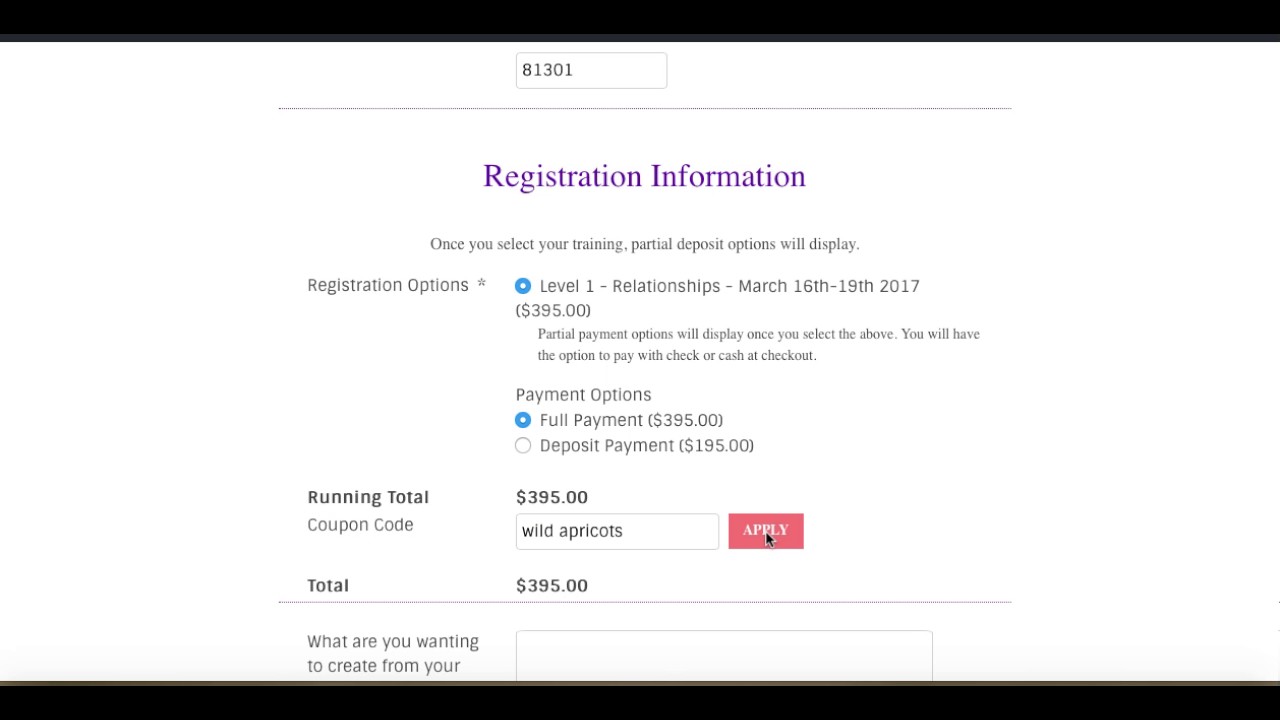This image is a screenshot taken from a webpage, although the specific website or company is unclear due to the absence of both the top header and footer. The screenshot features a solid black border at the top and bottom, with the remaining background in white. 

At the very top of the image, there is text in a gray font. Centrally positioned, the number "81301" is displayed, enclosed by a gray outline of a rectangle. Below this is a thin gray line serving as a divider. Positioned centrally under the line is the phrase "Registration Information" in a distinctive purple font. Further down, gray text indicates that partial deposit options will be shown once the user selects their training.

On the left-center of the image, various registration options are listed in gray font. These include:
- "Level 1, Relationships," scheduled for March 16-19, 2017, with a price of $395. It is noted in parentheses that partial payment options will become available once this option is selected.
- Users have the option to make payments via check or cash at the checkout. 

The payment options provided are:
- Full payment of $395
- Deposit payment of $195

Below the payment options, the running total is indicated as $395.

Adjacent to the payment information, there is a field labeled "Coupon Code." The text "wild apricot" is typed into this field, and it is enclosed within a small box. To the right of this box is a light pink button labeled "Apply" in large white font.

At the very bottom of the visible screenshot, the total amount of $395 is listed. Beneath this, a partial sentence reads, "What are you wanting to create from your," but the remainder of the text is cut off and not visible in the image.